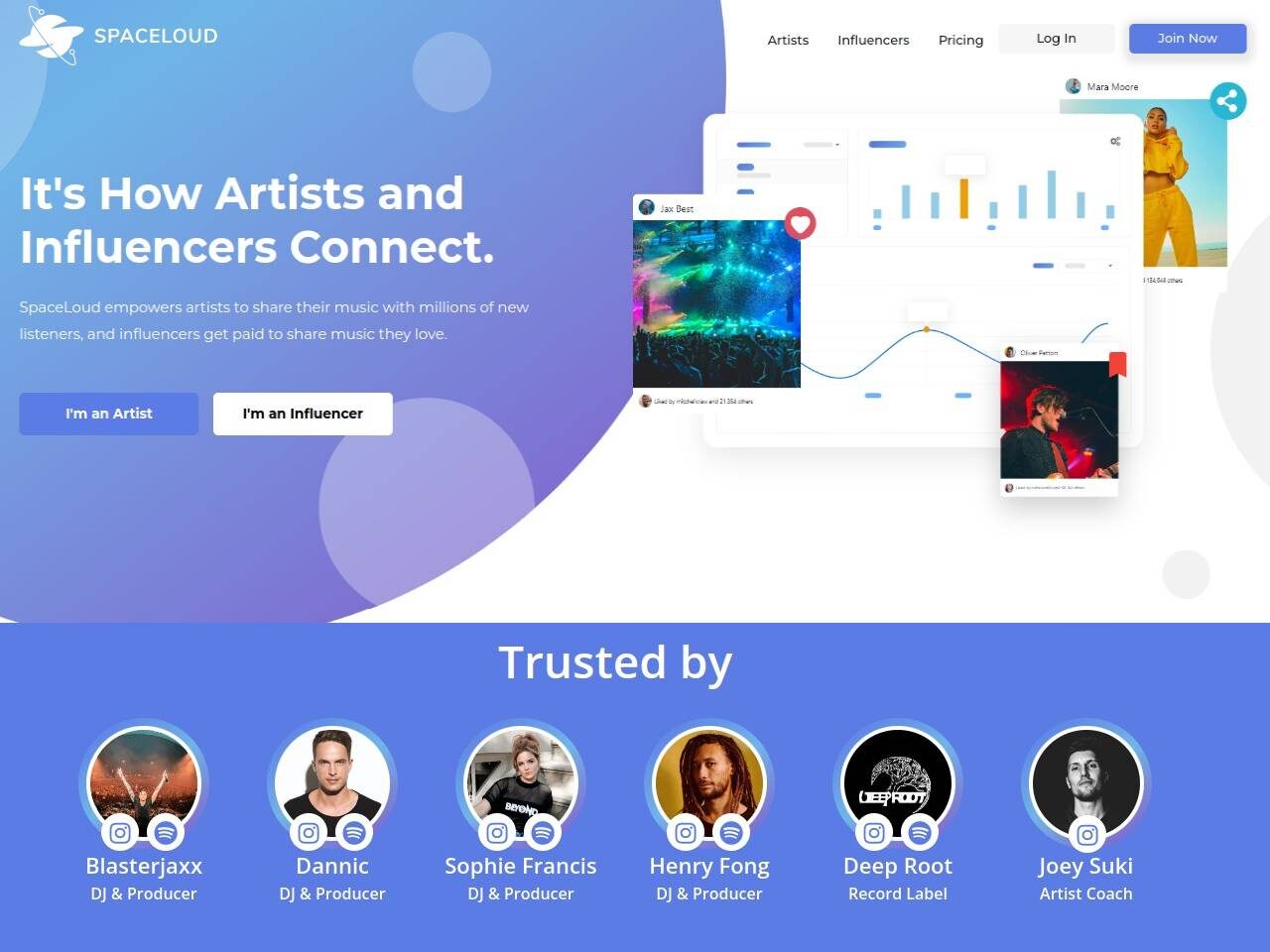Here is a cleaned-up and detailed caption for the image described:

---

In the upper left corner of the image is a graphic of a ring encircling a white line. Adjacent to this, the text "Space Loud" appears in white font. A couple of inches below, there is a larger white text stating, "It's how artists and influencers connect." Directly beneath this, in smaller white text, the description reads: "Space Loud empowers artists to share their music with millions of now listeners, and influencers get paid to share music they love." 

Below this text are two clickable options: a green box with the text "I'm an artist" and a white box with the text "I'm an influencer." 

At the bottom of the image, there is a blue square with white text that reads "Trusted by." Below this, the image features a series of circular photos.

- The first circle contains an image of a DJ with their hands raised, standing against a background that is red at the bottom and black at the top. Below this image, the text reads: "Blaster Jacks, DJ and producer."
- The second circle features a man with black hair and a black shirt. The accompanying text reads: "Danic, DJ and producer."
- The third circle displays a woman named Sophie Francis, who has brown hair and wears a black t-shirt with white text. The caption reads: "Sophie Francis, DJ and producer."
- The fourth circle is of Henry Fong, who is identified as a DJ and producer.
- The next circle features the name "Deep Root," which is identified as a record label.
- The final circle shows Joey Suki, noted as an artist coach.

---